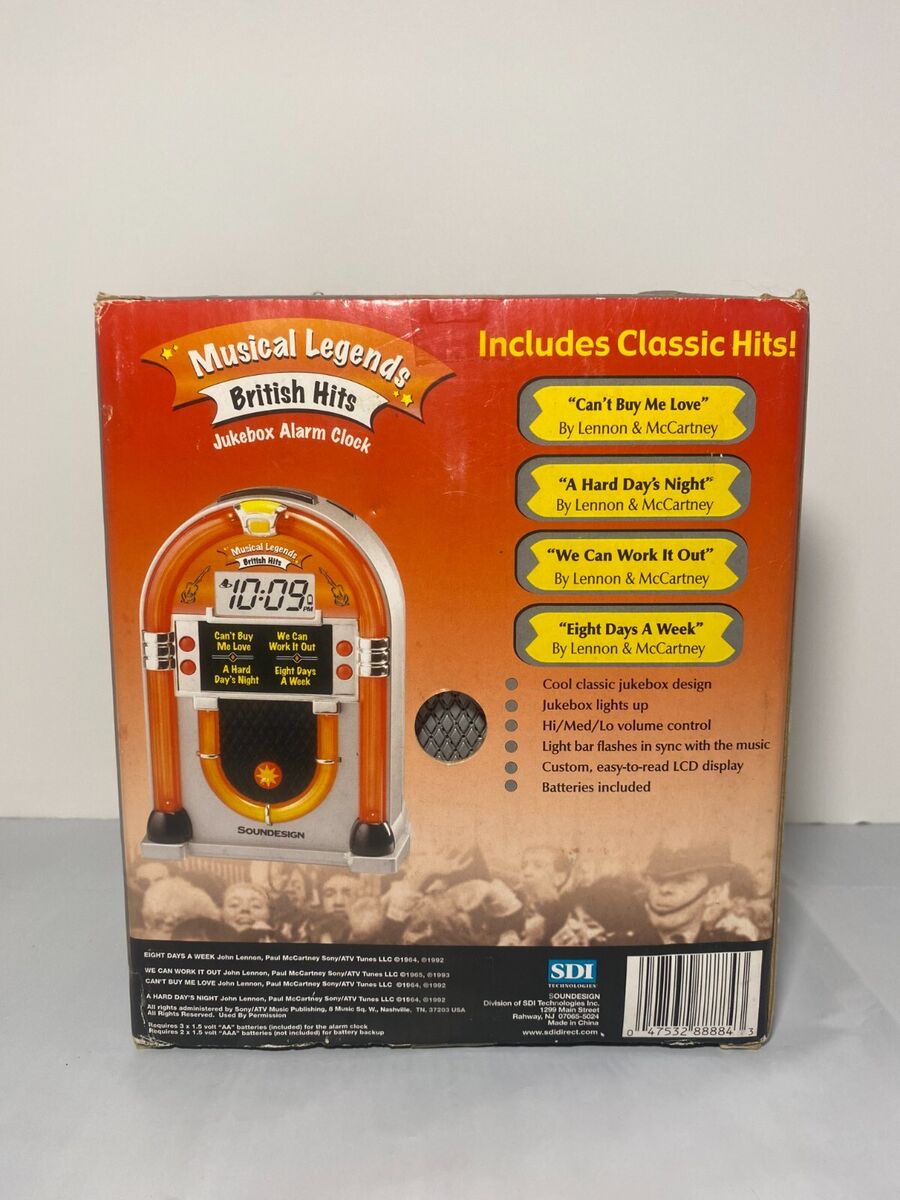The packaging for the Jukebox Alarm Clock, titled "Musical Legends British Hits Jukebox Alarm Clock," prominently features a nostalgic design. The box, which has a red background that transitions into orange and light pink hues towards the bottom, showcases an image of the gray and orange, curved-shaped alarm clock displaying the time 10:09. The upper left corner of the box announces the product name, while the right side highlights in yellow text that it "includes classic hits." Beneath this, four yellow text boxes with gray borders list the songs: "Can't Buy Me Love," "A Hard Day's Night," "We Can Work It Out," and "Eight Days a Week," all by Lennon and McCartney.

Further details include a bulleted list outlining the features of the clock: "Cool Classic Jukebox Design," "Jukebox Light Up," "High/MED/LO Volume Control," "Light Bar Flashes in Sync with the Music," "Custom Easy to Read LCD Display," and "Batteries Included." The center of the box has a cut-out revealing the waffle pattern of the speaker. At the bottom, a black and white photograph of excited fans contributes to the vintage theme, while a large horizontal black text box containing the UPC code is located on the lower right. The back of the box, primarily orange with gradient changes, repeats the product title and features in a similar layout. The box is seen lying on a gray floor against a white wall, with the design elements creating a visually appealing and detailed presentation of the Jukebox Alarm Clock.